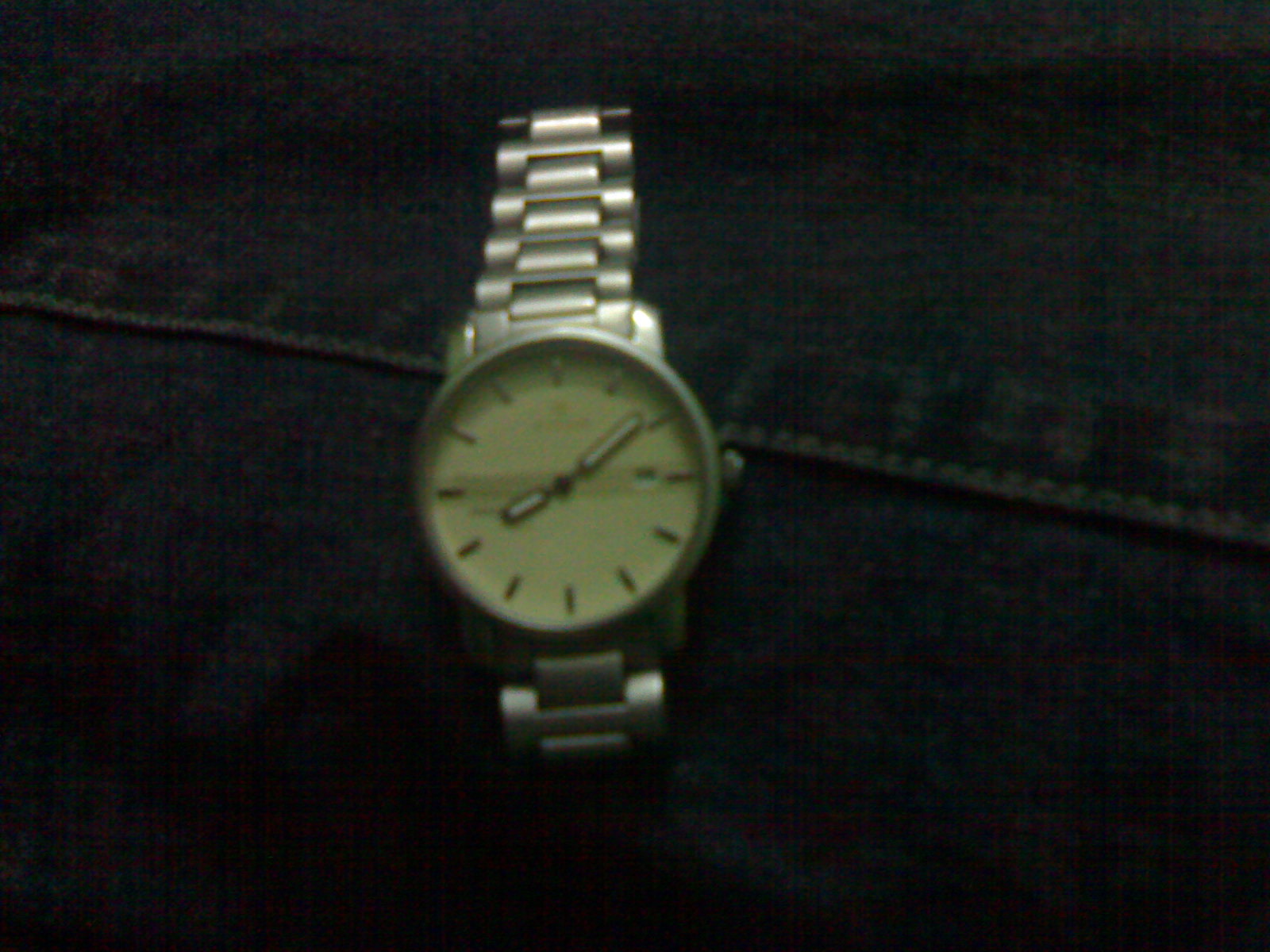A detailed close-up image shows a sleek, steel wristwatch with a circular beige watch face. The timepiece is elegantly designed, with a smooth, polished finish that gleams under the light. The lower part of the image captures a section of denim fabric, possibly from a pair of jeans, providing a contrasting texture and drawing attention to the watch's sophisticated simplicity.